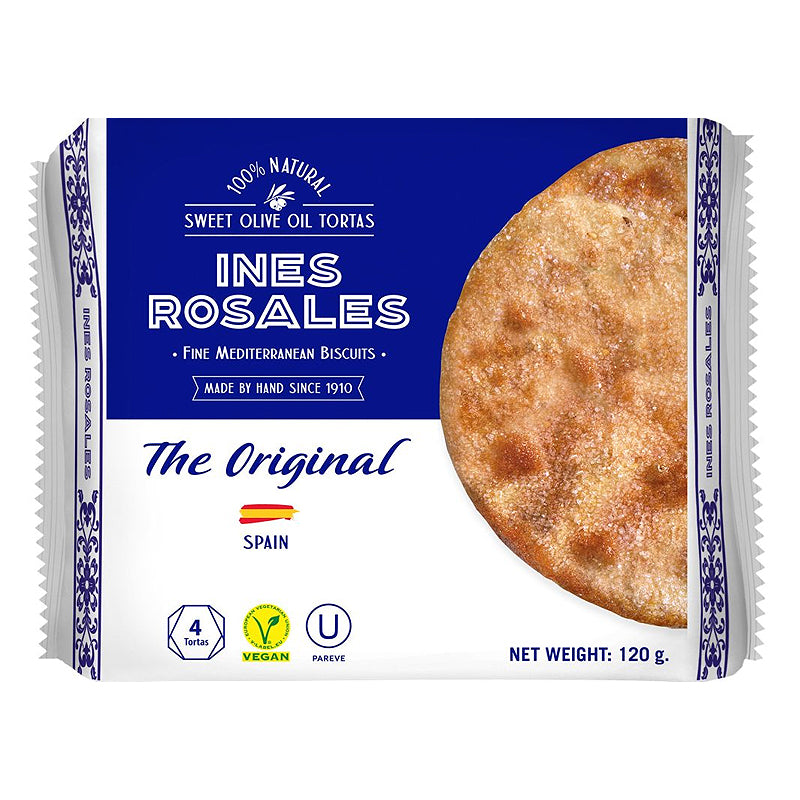This photograph showcases a package of Ines Rosales 100% Natural Sweet Olive Oil Tortas. The packaging, predominantly white with blue accents, features an elegant filigree design on the left and right sides, which fold over and lead to the vacuum-sealed, crimped ends. A blue area dominates the top half, containing white text that reads "100% Natural Sweet Olive Oil Tortas" in a large, bold font, along with "Ines Rosales," the brand name. Below this, in smaller white text, it states, "Fine Mediterranean Biscuits Made by Hand Since 1910," and in blue cursive, "The Original."

The bottom half of the package is white, displaying a picture of a golden-brown, round flatbread sprinkled with salt. There's a small Spanish flag indicating the product's origin, along with the word "Spain." Four symbols line the bottom: the first indicating "Four Tortas," the second highlighting "Vegan" in yellow and green, the third featuring a circled "U" accompanied by the term "Parve," and the fourth denoting the net weight of 120 grams. This artisanal product, from Spain, is marketed in several major retailers, including Whole Foods.